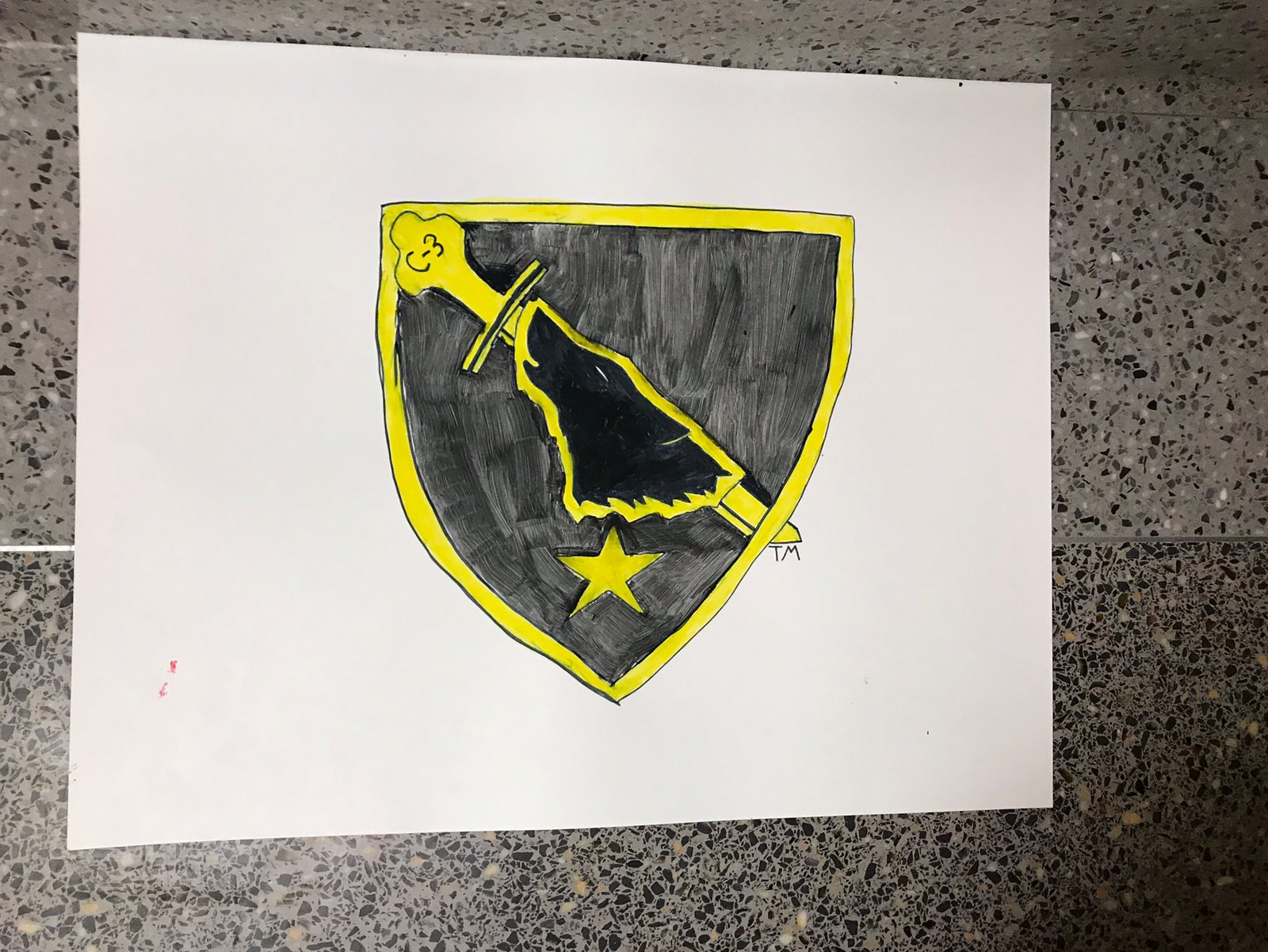A hand-drawn image is displayed on a white printer paper sheet. The drawing features a yellow star with a yellow outline, dominating the design. The star's center is filled with various shades of dark gray, creating a textured look. At the very center of the star, there is a striking black area, possibly representing a focal point. A yellow emblem, resembling the shape of a narrow broom or a sword, is also incorporated into the design. The paper rests on what appears to be a granite kitchen countertop or possibly a gray, speckled floor surface, hinting at a casual, everyday environment where the drawing was made.